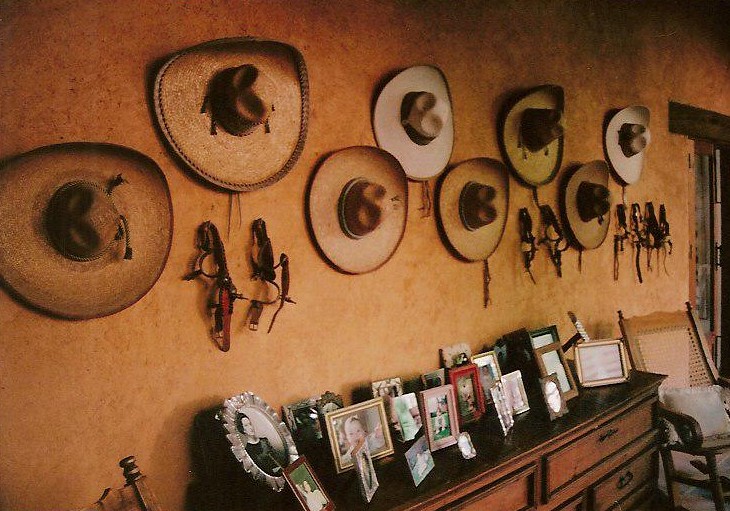The image showcases a cozy, Southwestern-inspired room with an inviting, homey atmosphere. The pale orange stucco wall serves as the backdrop, adorned with a zigzag display of eight woven sombreros. Beneath these hats, some authentic cowboy spurs dangle, adding to the rustic charm. A mid to dark brown wooden dresser stands against the wall, partially cut off but clearly visible, with a collection of approximately 20 framed photographs on its top surface. These frames vary in size and material, with both wood and metal finishes, and they predominantly feature images of family members, including older relatives and even a baby. To the right of the dresser is a wooden rocking chair with a wicker back and a white throw pillow, completing the inviting scene.